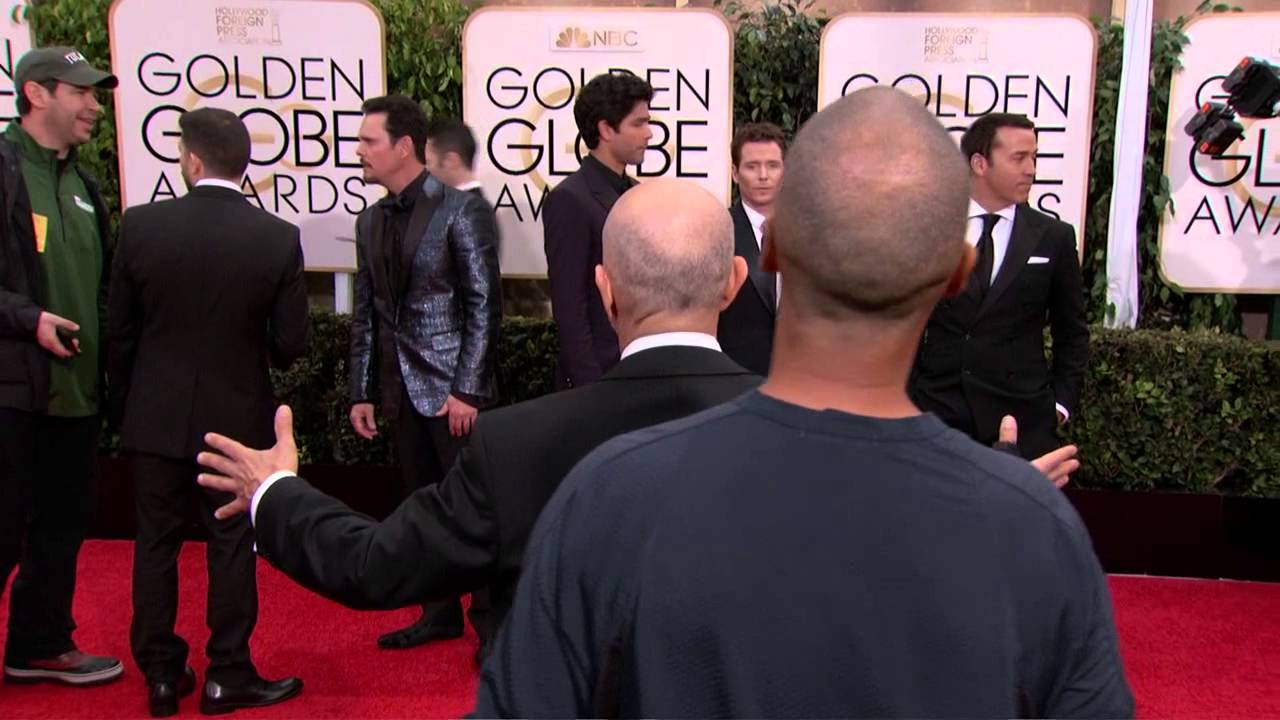This detailed image captures the red carpet scene at the Golden Globe Awards. The iconic red carpet stretches before a backdrop of perfectly squared-off green hedges, above which four prominently displayed signs read "Golden Globe Awards" in bold black lettering, one of which includes the distinctive NBC peacock symbol. In the upper right of the image, lighting setups are partially visible, enhancing the ambiance of the event. Several attendees, likely actors and other figures linked to the awards, are present, distinguished by their attire. Most are in dark suits and ties, with the notable exception of a man in a shiny blue tuxedo jacket. In contrast, another prominent figure in the foreground is dressed casually in what appears to be a bluish sweatshirt or long-sleeve shirt. Other individuals include a man conversing in a green hat and polo, another in a traditional black suit, and across the scene, composed groups engage in conversation, capturing the bustling, anticipatory atmosphere of the pre-show red carpet event.